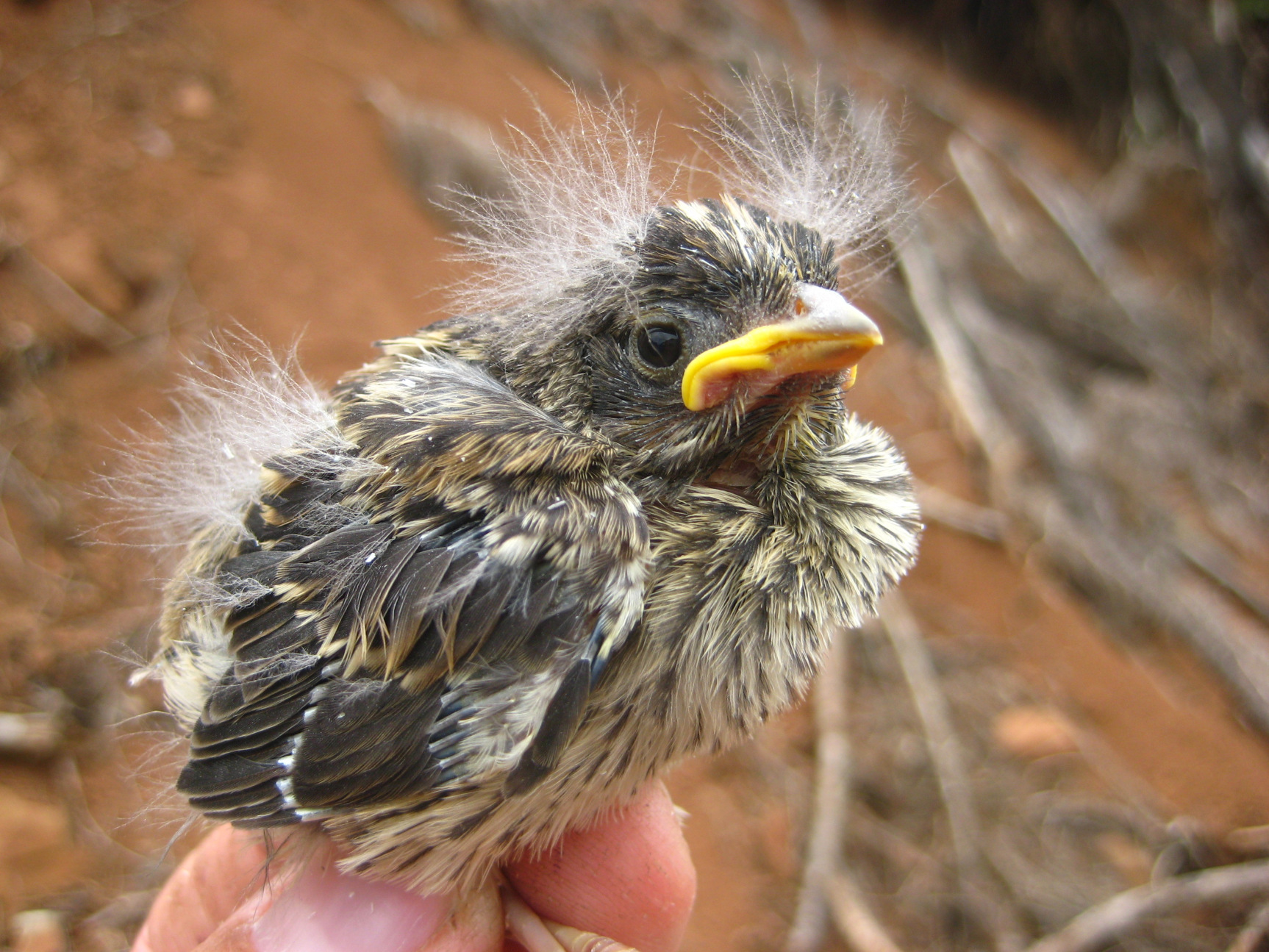The image depicts a small baby duck, identifiable by its large yellow bill and soft, partially developed feathers. The duckling has a mix of white and black coloring; its wings are predominantly black with white markings while its stomach and chest are mostly white with some black markings. Notably, it has white, long, fuzzy feathers around the area where its ears would be. The bird's eye is visible and it appears calm, gazing towards the camera. Held gently by a person's hand, three fingers are seen supporting its back and legs. The background, although out of focus, reveals an outdoor scene with dark mud and some leafless sticks and branches, suggesting a fall or winter setting. The bright daylight ensures the image is clear and well-lit, emphasizing the delicate features of the duckling's soft, cottony feathers.